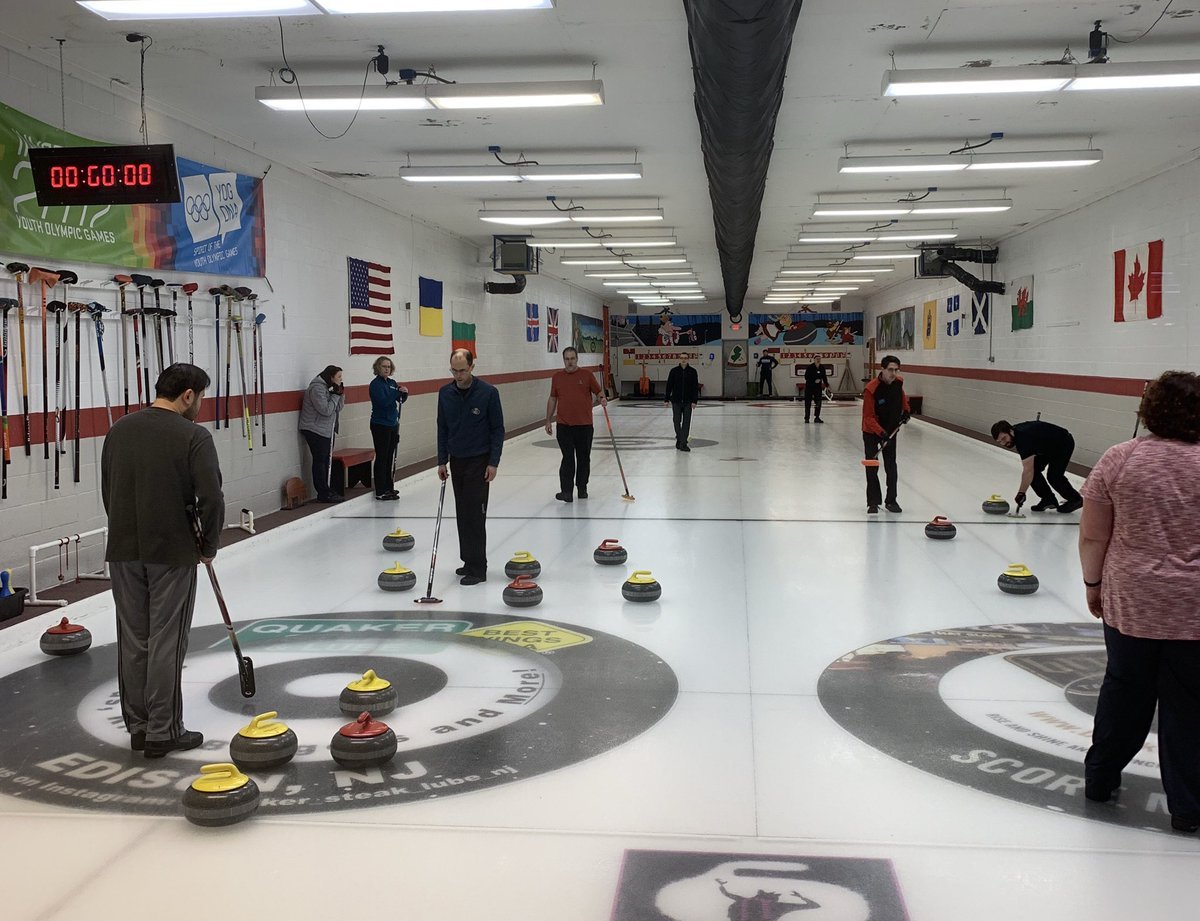The image captures a lively scene inside a curling arena featuring two lanes occupied by individuals engaged in a game of curling. The floor is marked with large circles and grid patterns commonly seen in curling rinks. Players, both male and female, are focused on the game, holding curling brooms to strategically sweep stones across the gleaming ice. The curling stones are vividly colored in yellow and red, scattered across the playing surface. Adorning the walls are numerous international flags, including those of Canada and the United States, and curling brooms are neatly hung along the left side. A digital timer hangs from the ceiling, currently displaying zeros, illuminated by the surrounding neon and white fluorescent lights. The soft white bricks of the walls add a gentle contrast to the vibrant action below. Above the scene, a long black pipe runs across the ceiling, adding a structural element to the energetic environment. There is also a prominently displayed banner reading "Youth Olympic Games," partially obscured by an LED sign, reinforcing the arena's connection to international sports and youth development.